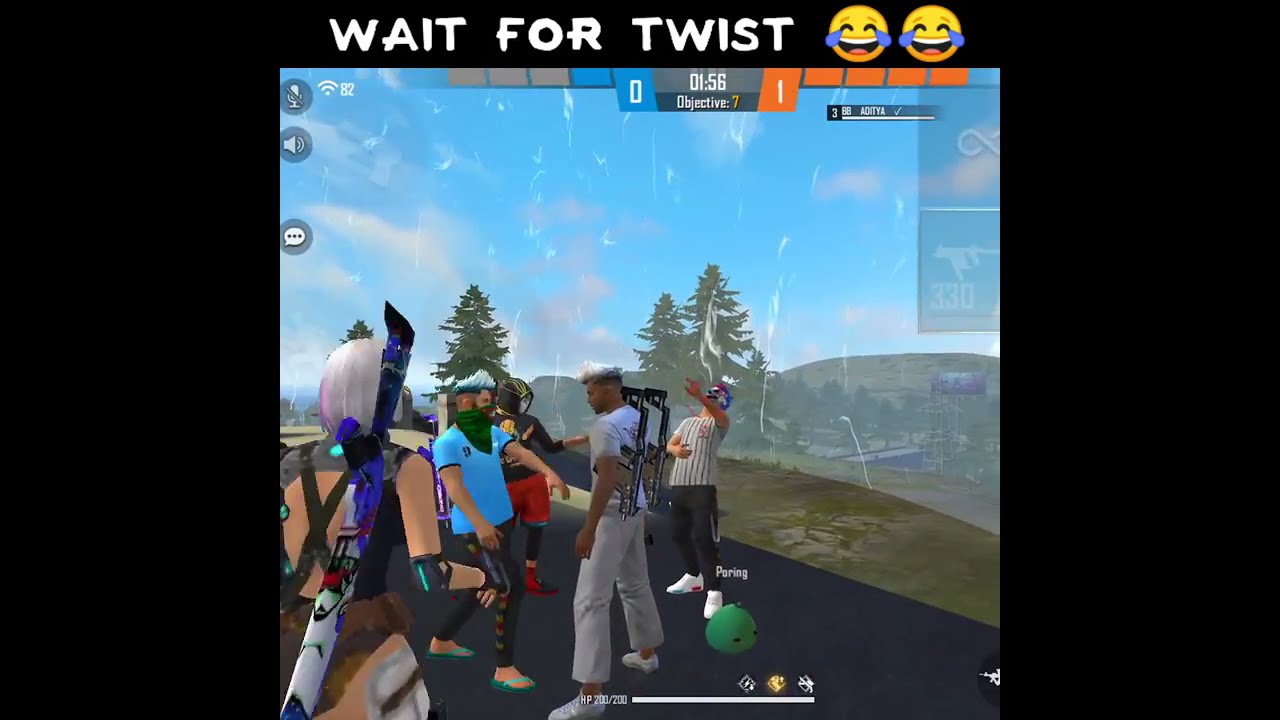The image appears to be a cartoonish screenshot from a three-dimensional sports or adventure video game. It features a vibrant, outdoor scene with a diverse group of five characters standing on what appears to be a street amidst buildings, mountains, and trees under a blue sky with clouds. The backdrop hints at rain. Each character dons colorful and eclectic outfits, including accessories like masks or bandanas. They each have what seem to be jetpacks or similar gear on their backs. At the top of the screen, white text on a black background reads "wait for twist" along with two laughing-crying emojis. The atmosphere is lively, with characters seemingly laughing and pointing at the sky, suggesting camaraderie and shared amusement. Minimal text is seen, including "156" and "objective 7," alongside an HP indicator at the bottom showing "200/200."